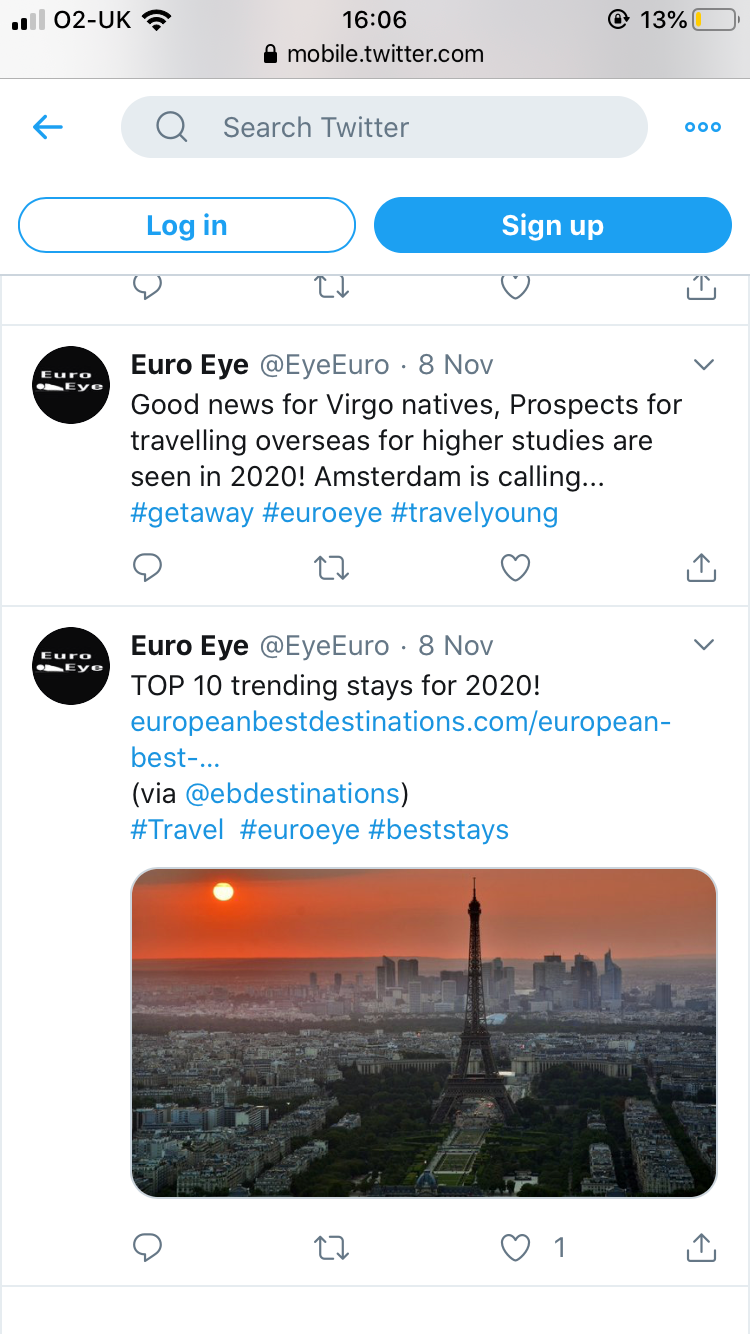The image captures the screen of a mobile phone displaying a page from mobile.twitter.com. In the top-left corner, the signal strength bars, the "O2 UK" network name, and a Wi-Fi indicator with a strong signal are visible. Centrally located on the grey top panel, the clock reads 16:06, and the URL mobile.twitter.com is displayed, indicating the active site. On the right-hand side, the battery icon shows a remaining charge of just 13%.

Below the URL section, the Twitter interface features a search bar labeled "Search Twitter." Directly beneath the search bar, there are two buttons: a white "Login" button on the left and a blue "Sign Up" button on the right. 

Further down, two news items from EuroEye are displayed. The first news headline reads, "Good news for Virgo natives. Prospects for traveling overseas for higher studies are seen in 2020. Amsterdam is calling." The second news item, also from EuroEye, highlights "Top 10 trending stays for 2020," and includes a clickable link to europeanbestdestinations.com in blue lettering, along with hashtags such as #travel, #EuroEye, and #beststays.